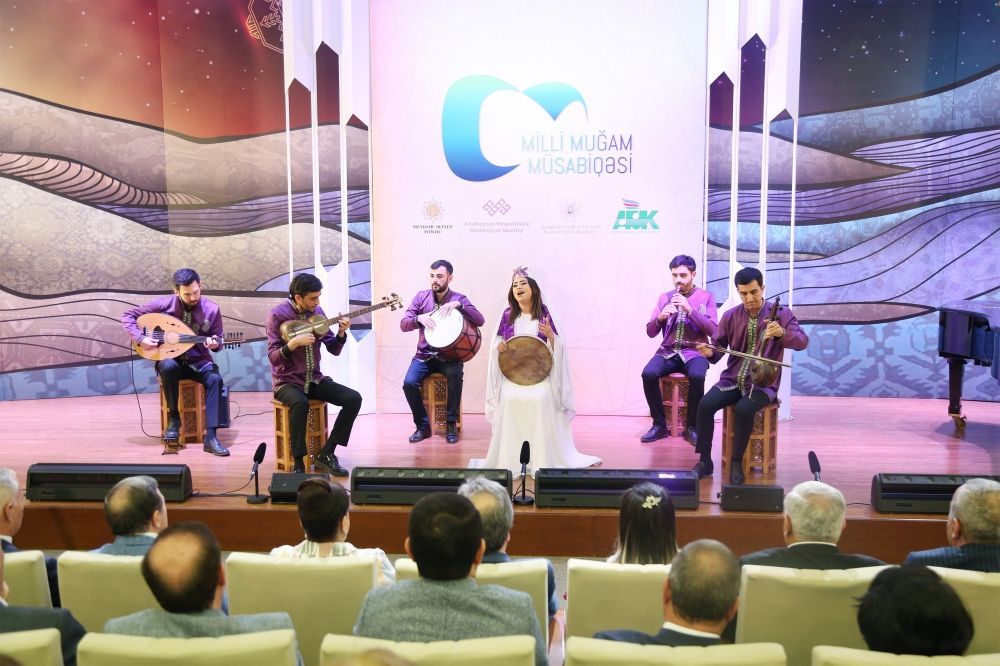The image showcases a photorealistic performance scene featuring a Middle Eastern or South Asian music ensemble. The stage is adorned with a vibrant, stylized backdrop of purple mountains and other colored hills, creating an elaborate and dynamic setting. Central to the performance is a female vocalist, dressed in a white gown with a purple shawl, flanked by five male musicians all wearing purple tops and dark trousers. Each musician is seated on brown stools, playing unique instruments including guitars, a grand piano, drums, a flute, and a violin-like string instrument. Behind them, a sign reads "Milli Mugam Musa Bukiwasana," indicating the title of the event and listing four sponsors underneath. In the foreground, two rows of audience members sit in gold cushioned chairs, predominantly men with a few women, attentively watching the performance under the glow of stage lights.